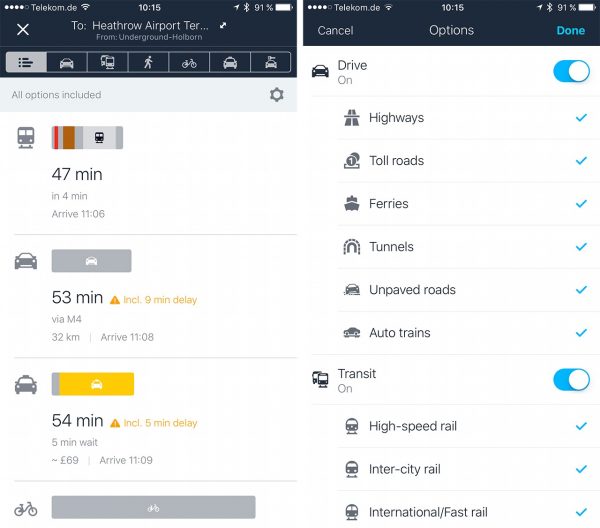**Image Description:**

The image comprises two screenshots, both displaying the time as 10:15 AM and the battery level at 91%, with a white background.

- **First Screenshot:** 
    - A detailed route planning interface showing possible modes of transportation from "Carthrow Airport" to "TER... underground coal barn."
    - Icon representations for various modes: car, bus, walking, bicycle, taxi, and rental car options.
    - A blue rectangular button labeled "Include All Options" accompanied by a settings icon.
    - Travel durations specified for each mode:
        - Bus: 47 minutes
        - Car: 53 minutes
        - Taxi: 54 minutes
    - An attention sign indicating an included delay:
        - Bus: 5-minute delay
        - Car: 9-minute delay
    
- **Second Screenshot:** 
    - Displaying options to customize driving routes with "Cancel" on the left and "Done" highlighted in blue on the right at the top.
    - "Drive On" option is toggled on.
    - Route preferences with check marks next to:
        - Highways
        - Toll Roads
        - Ferries
        - Tunnels
        - Unpaved Roads
        - Auto Trains